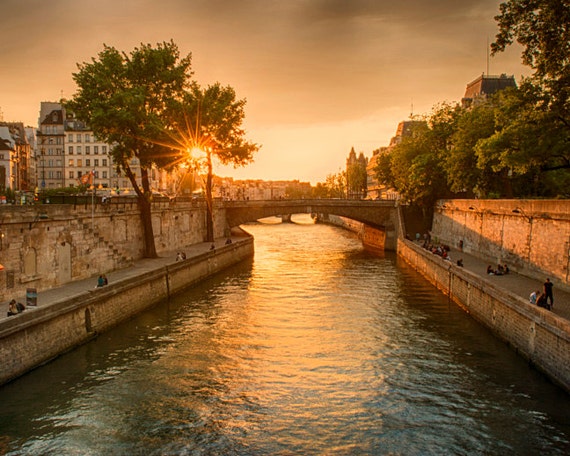The image depicts a serene, likely European town at sunset, possibly resembling Venice, Florence, or Paris. A river, with greenish-brown water, flows through the center of the scene, flanked by brick or cement walkways on either side. These walkways are lined with green trees, occasional trash cans, and various people either walking or sitting, predominantly visible on the right side. A prominent bridge spans the river, connecting both sides, and adding to the charm of the scene. The background is adorned with an assortment of buildings, including white structures with numerous windows and darker buildings topped with spires. The setting sun casts a shimmering reflection on the water, enhancing the tranquil atmosphere of this picturesque locale.